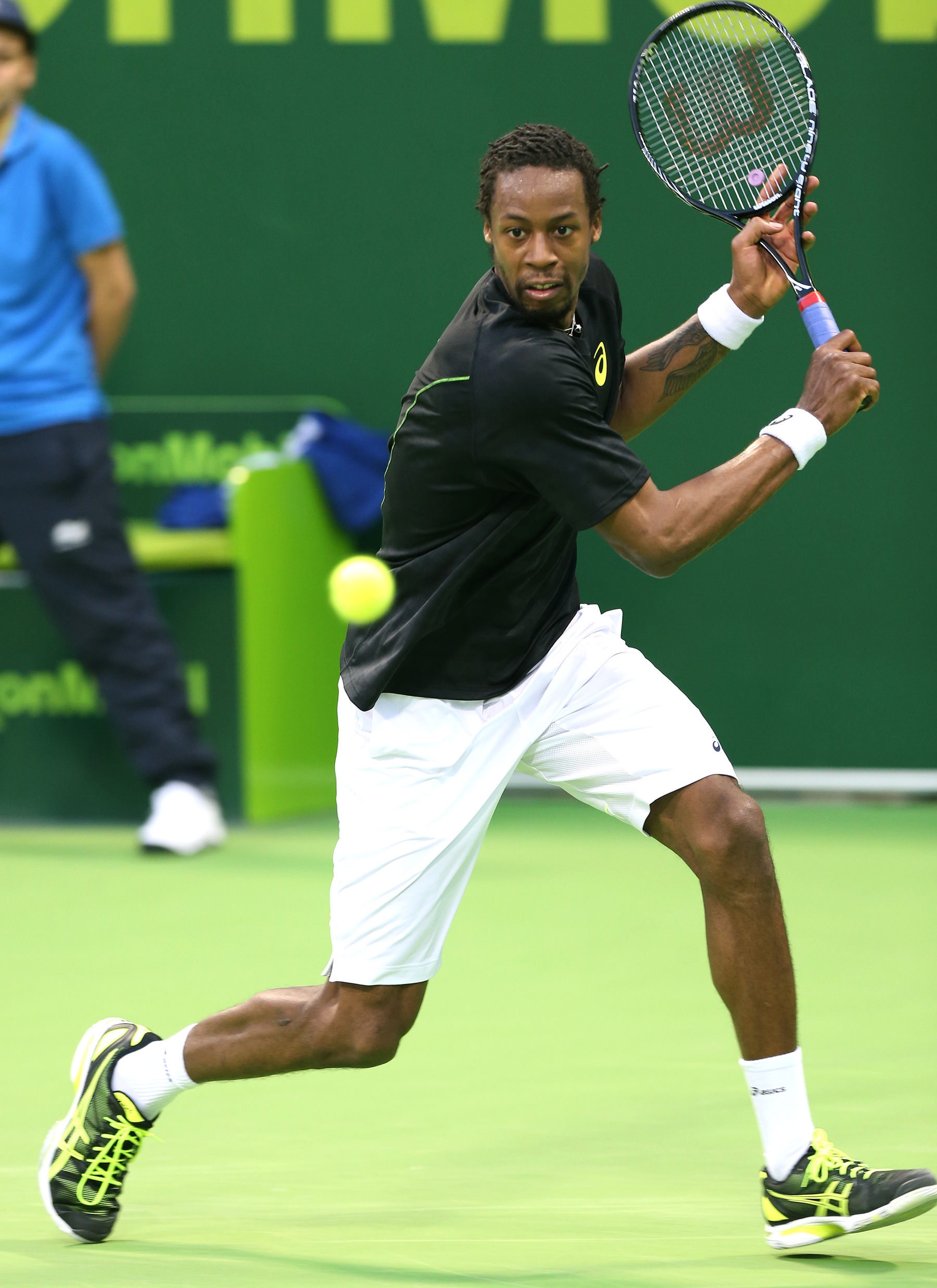In this photo, a young African-American man, likely in his 20s or 30s, is captured mid-motion on a tennis court. He is lunging to his left, ready to execute a backhand shot towards a tennis ball suspended in midair, directly in front of him. His upper body twists with determination as he prepares to swing his racket, held with his right hand while his left hand grips the neck. He is dressed in a black polo shirt featuring a yellow ASICS logo on the left side of his chest, paired with white shorts. His attire is complemented by white wristbands, white socks that rise above his ankles, and black-green-white sneakers. His hair is styled in short, rolled sections. The action unfolds on a green tennis floor, against a solid green wall. In the background, to the left, another man dressed in a white and blue top with black pants stands facing the camera, with one arm positioned behind his back.